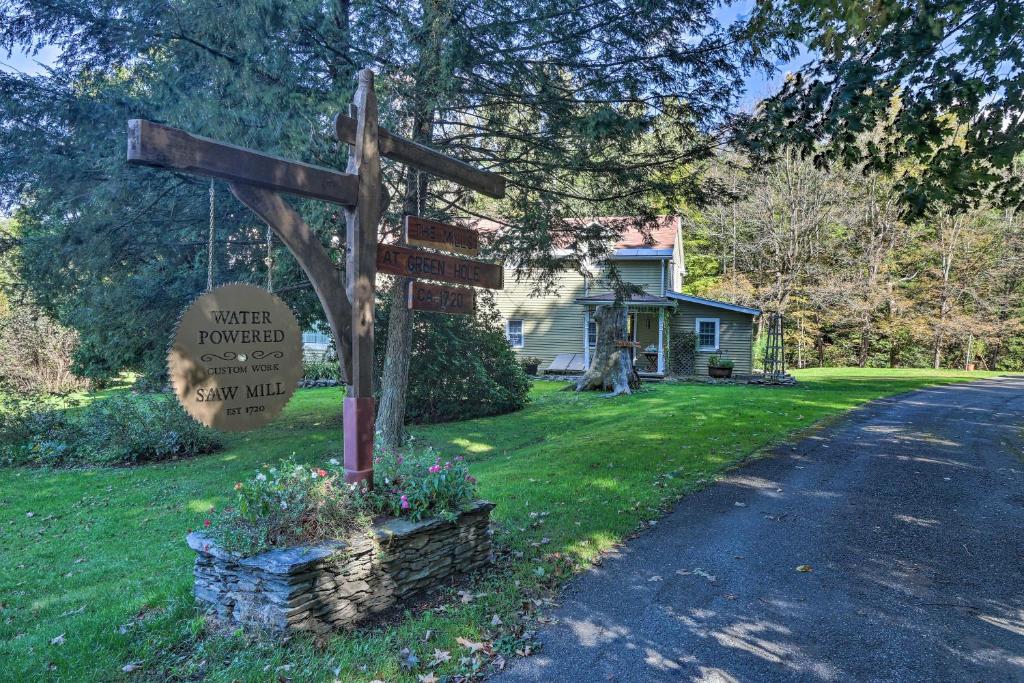The photograph captures a picturesque countryside scene in the middle of a sunny day, showcasing a historic location. A charming greenish pea-colored farmhouse with a red roof is nestled amidst lush green lawn and enveloping woodland. The house is accentuated by sunlight dappling through the trees, contributing to the bucolic setting. 

On the right side of the image, a blacktop driveway bordered by foliage invites the viewer into the serene property. In the foreground, prominently displayed, is a vintage sign made from an old saw blade with serrated edges, hanging from a wood post over a stone planter filled with vibrant flowers. The sign reads, "Water Powered Custom Work Sawmill Established 1720." Additional wooden planks with various directional instructions hang beneath the primary sign. This rustic ensemble, set against the backdrop of the modern-yet-historic farmhouse and the beautiful rural landscape, captures the essence of timeless craftsmanship and the enduring beauty of countryside life.